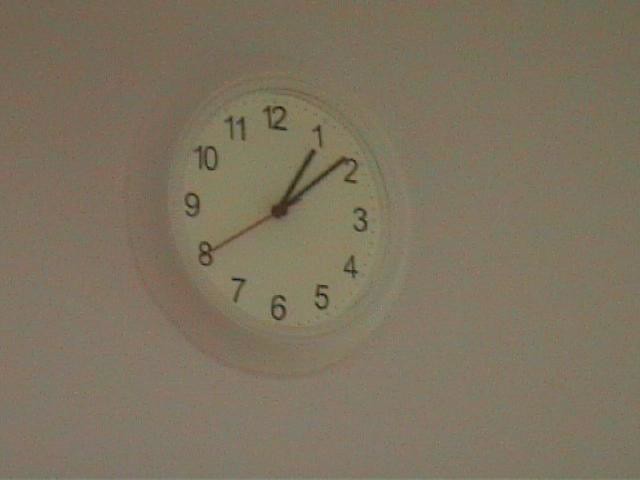"The image depicts a centrally positioned, circular clock set against a plain white background. The image quality is notably poor, characterized by a low resolution, significant blurriness, and pixelation. The clock's frame is white, complementing the black numerals that are arranged in a counterclockwise direction, starting from 12 at the top and progressing leftward to 11. The clock face features two black hands for the hours and minutes, and one red hand for the seconds. The simplicity of the background and the distorted focus draw attention solely to the clock, emphasizing its unique counterclockwise numbering."